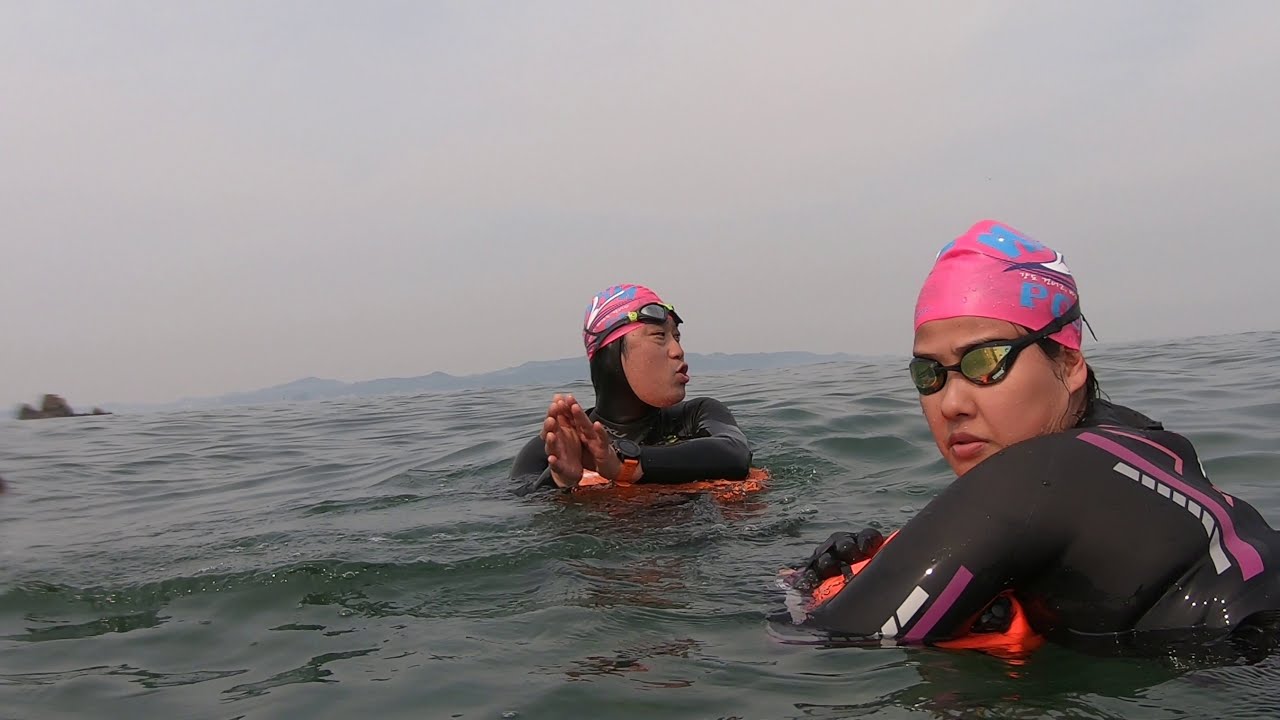The full-color photograph, taken during the day amidst an overcast, gray sky, captures an outdoor scene set in a large body of water, likely the ocean due to the visible waves. In the foreground are two swimmers, possibly of Asian or Pacific Islander descent, wearing identical black wetsuits adorned with purple, pink, and white designs, complemented by pink swimming caps with blue and white patterns. They each wear goggles, though the man has his positioned on his forehead, while the woman has hers over her eyes and is also wearing gloves. Both swimmers are holding an orange flotation device. The man, centrally positioned and gazing off to the right, has his hands in front of him, whereas the woman, situated more to the right, faces the camera directly. In the backdrop, there is raised land and a rocky outcrop on the left side, further emphasizing the open water setting.